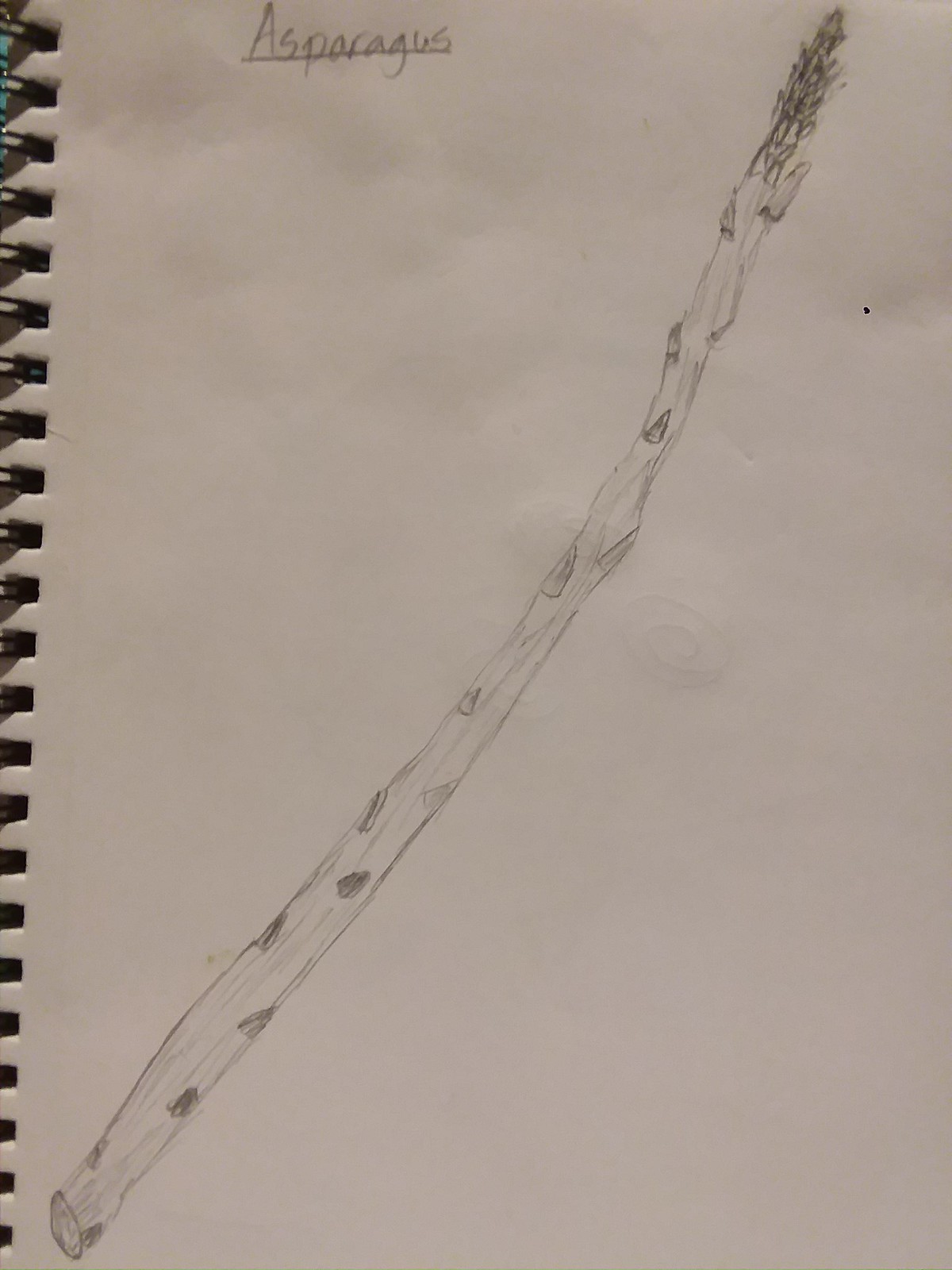The image depicts a simple pencil sketch of a piece of asparagus in a spiral-bound sketchbook. The asparagus, extending diagonally from the bottom left to the top right, is rendered with modest detail, showing more shape and form than a young child might produce. The stalk features little leaves sticking out, contributing to its recognizable structure. Above the sketch, "asparagus" is written in simple print and underlined. The sketchbook's page, slightly yellowed and grayish, shows imprints of adjacent writings. The sketchbook is open, and the photograph captures the overhead view with the holes in the binding being small squares rather than circles. The image is somewhat dim, indicating a less brightly lit environment.